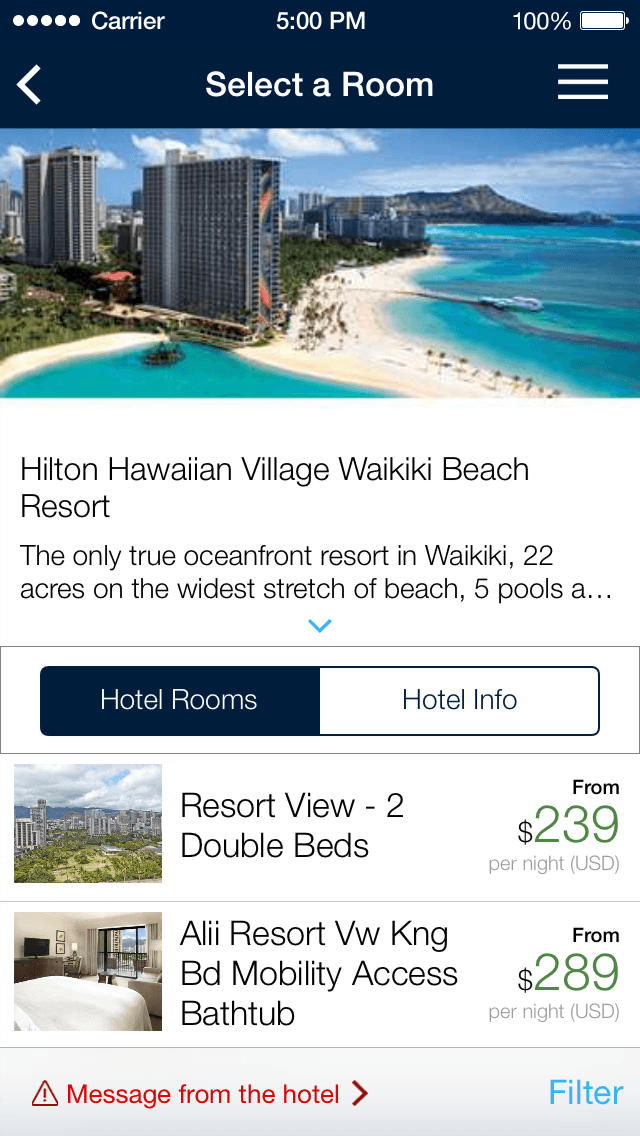This screenshot depicts a mobile-optimized room booking website. The screenshot is taken in portrait orientation, indicating it was captured on a mobile device. At the top of the screen, there is a header displaying "Select a Room." Just below the header, an image showcases the stunning Coastline City, featuring towering skyscrapers, a sandy beach, and distant mountains.

Further down, the text "Hilton Hawaiian Village, Waikiki Beach Resort" identifies the specific location. The description highlights the resort as the "only true oceanfront resort in Waikiki," spanning 22 acres along the widest stretch of beach. The description mentions several amenities, including five pools, but is cut off with an ellipsis, implying additional information can be revealed by scrolling down.

Below this section are two interactive buttons labeled "Hotel Rooms" and "Hotel Info," with "Hotel Rooms" currently highlighted. Under the highlighted tab, there are two room options available for booking:

1. "Resort View, Two Double Beds" starting at $239.
2. "Ali'i Resort View, King Bedroom, Mobility Access with Bathtub" starting at $289.

The design clearly prioritizes user-friendly navigation and accessibility, allowing potential guests to effortlessly explore and book accommodation.